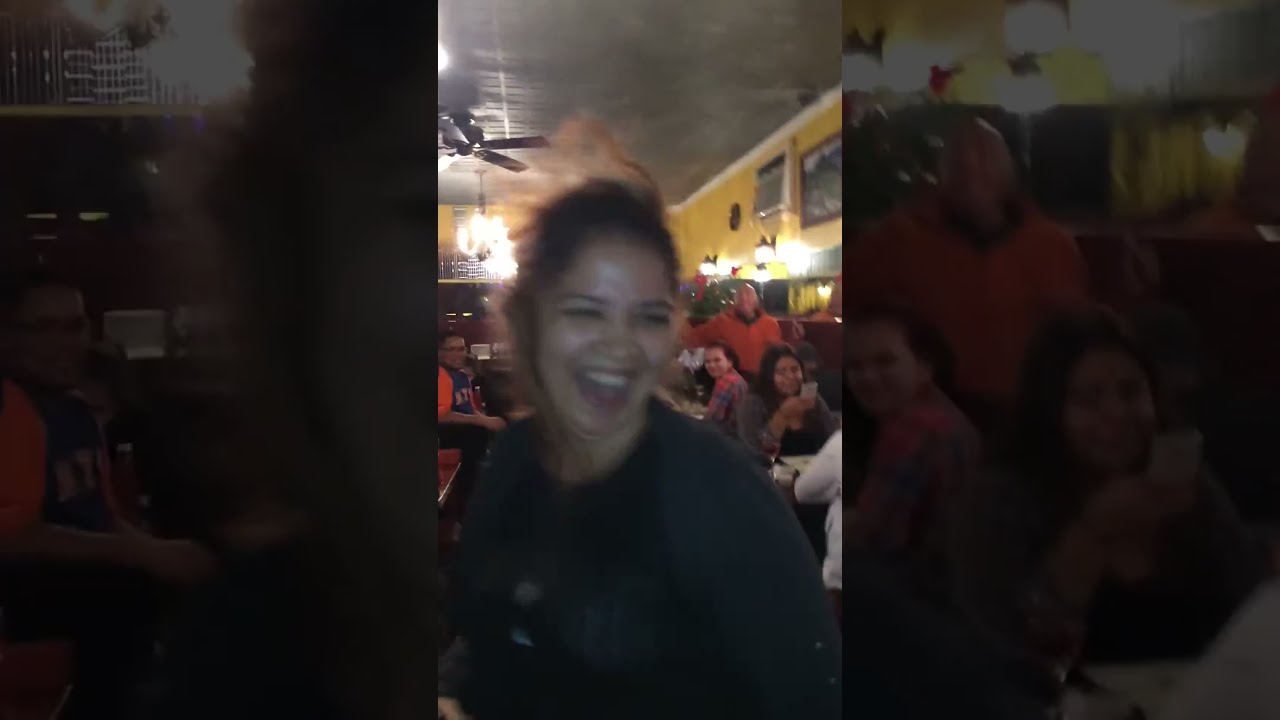In this detailed photograph, four people are seated at a large, brown, rectangular wooden table at a restaurant, appearing to enjoy a festive gathering. The woman closest to the camera, positioned on the right side in the foreground, has short dark hair and is holding a black microphone up to her mouth, seemingly singing. She is a white woman wearing a black sweater over a light-colored shirt. On the table, there are various items, including a silver Corona bucket containing a bottle of champagne, Corona beer bottles, napkins, and other miscellaneous items.

Seated across from her at the table are three people: a woman in a red dress with short brown hair and clapping hands, a woman in a black dress also clapping, and a man with short dark hair wearing a blue button-down shirt. They are all seated on a cushioned brown bench. Behind them, the wall features a large painting within a rectangular gold frame, depicting a park scene with people walking on a path. The overall scene is framed within two vertical black bars, giving it a formal presentation.